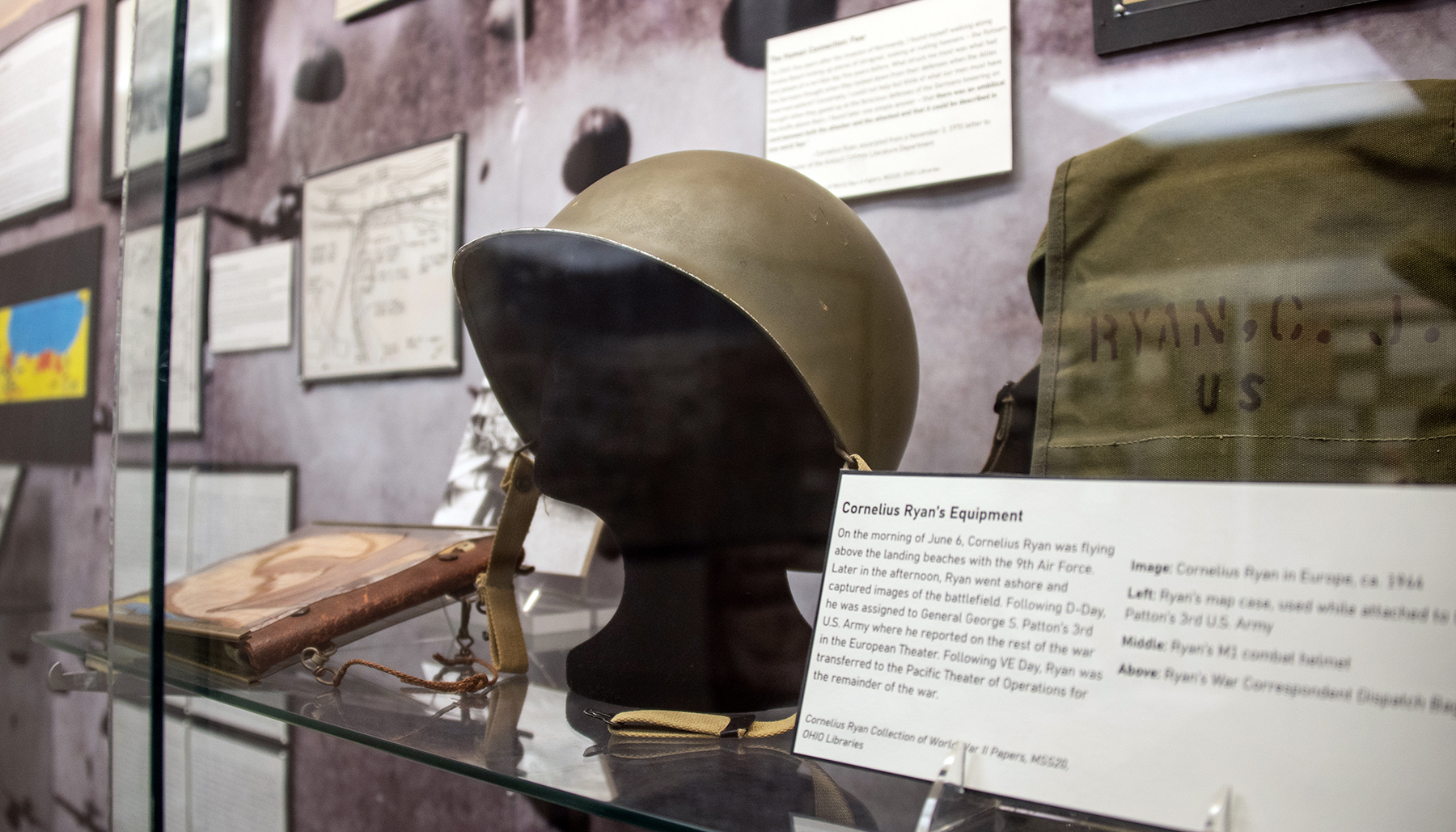In this detailed photograph taken within a museum or private collection, a variety of old antique military relics are showcased, encased in protective glass. Central to the display is an army green soldier's helmet perched on a black mannequin head, which is oriented towards the left. To the right of the helmet, there is an olive green military bag emblazoned with the name "Ryan C.J. U.S." Below the bag and the helmet, resting on a glass shelf, is a small white informational card that reads "Cornelius Ryan's Equipment." This card details Cornelius Ryan’s significant contributions during WWII, mentioning his activities on D-Day with the 9th Air Force, his subsequent assignment with General George S. Patton's 3rd U.S. Army, and his later transfer to the Pacific Theater of Operations.

To the left of the helmet, an old leather-bound log journal, possibly carried and written in by Ryan, is positioned. The wall behind the display, featuring a mottled maroon hue, is adorned with framed photographs, printed signs, and other historical documents, which add historical context to the artifacts. This arrangement of relics, carefully preserved and displayed, offers viewers an insightful glimpse into Cornelius Ryan's wartime experiences and equipment.